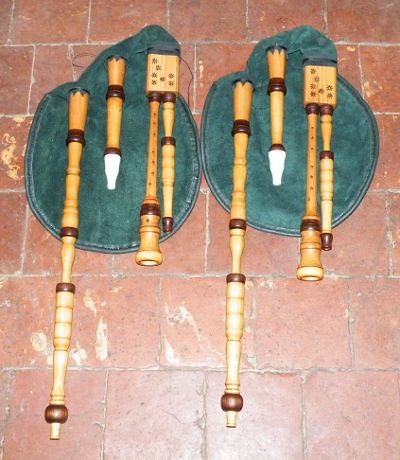In this photograph, we see two sets of wooden bagpipes resting symmetrically on a dark red brick surface that shows signs of wear with various scratches and etches. Each bagpipe consists of a deflated green leather bag that lies flat, resembling the shape of a ping-pong paddle. Attached to these bags are multiple wooden components that collectively resemble pipes or flutes. These attachments vary in length, with some being more than double the size of the others. They feature intricate carvings and darker brown rings which might either be decorative or separate wooden sections joined together. Each set has a large opening where you'd blow to produce music. Additionally, holes are visible on some of the pipes, similar to those found on flutes. All the components are placed atop round green felt pads to protect both the bagpipes and the surface beneath from scratches. The central subject of this image is clearly these two intricately crafted bagpipes placed on a vintage, well-worn brick floor.